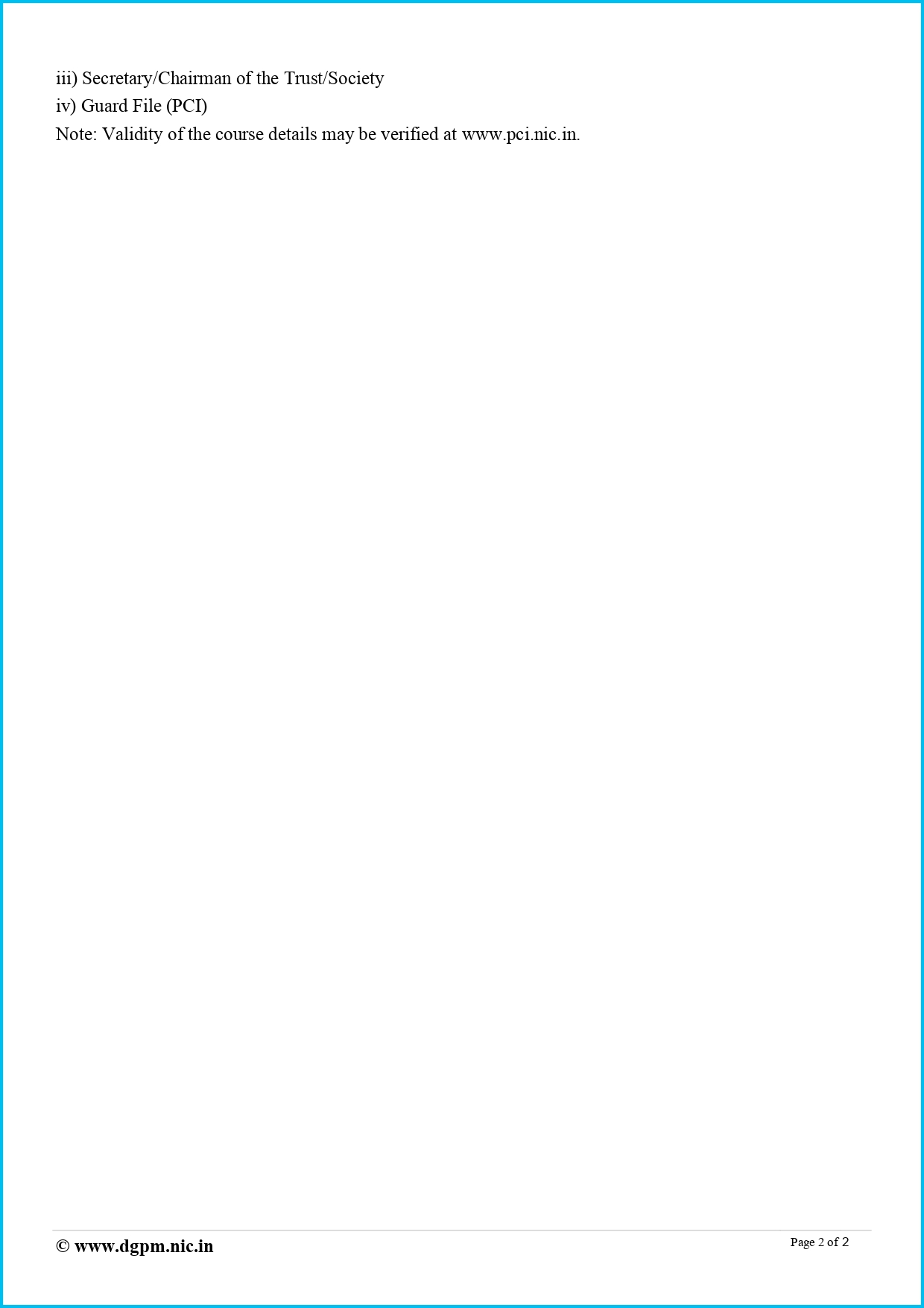The image resembles a large sheet of paper with a predominantly white background. The edges of the paper are highlighted by a bright blue border. In the upper left corner, there are Roman numerals "III" followed by the text "Secretary, Chairman of the Trust/Society." Below that, the numeral "IV" is listed, corresponding to "Guard File" with "PCI" in parentheses. Underneath this, a note reads: "Validity of the course details may be verified at www.pci.nic.in."

The majority of the page remains blank except for the information concentrated at the bottom. In the bottom left corner, there is a small circle with a "C" inside it, followed by the text "www.dgpm.nic.in." On the bottom right corner, it states "Page 2 of 2." At the very bottom of the page, a thin gray line runs horizontally, separating this section from the rest of the content.